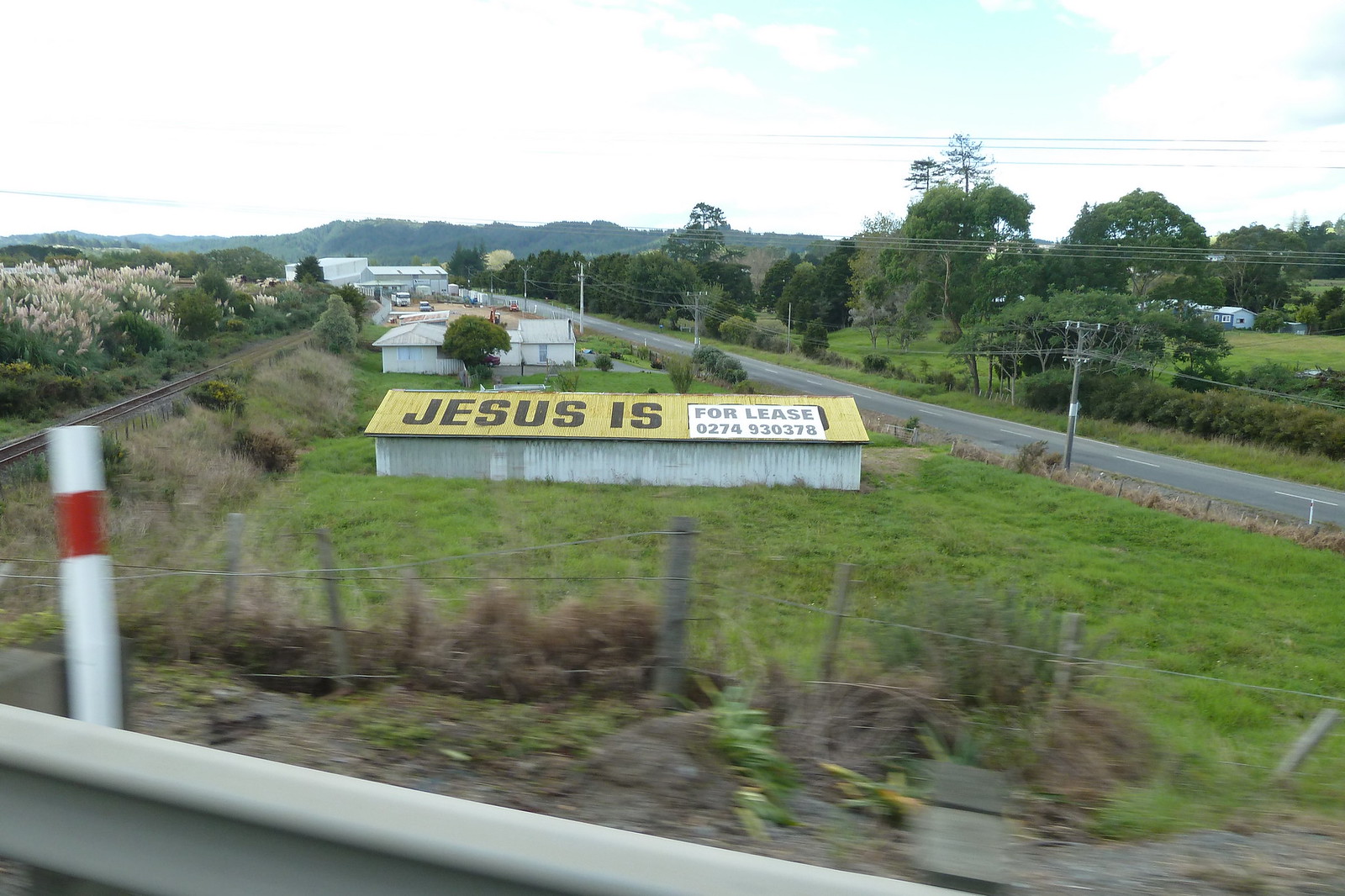In this vibrant summer photograph taken from a moving car, a white building with a bright yellow roof stands prominently in the center. The roof features large black capital letters spelling "JESUS IS," partially obscured by a white and black "FOR LEASE" sign, suggesting a peculiar message: "Jesus is for lease." The sign includes the phone number 0274 930378 for inquiries. The building, which has the appearance of an old shed or mobile home, sits amidst a lush green field, contrasting with its stark architecture. Surrounding the building, there are power lines and a strip of other buildings, hinting at a main road nearby.

In the foreground, a highway guardrail and a fence with wooden poles mark the edge of an overpass or roadside barrier, adding depth to the scene. The guardrail is accompanied by some dark brown dirt and a pole with white and red markings. Past the green field, additional white buildings and green hills stretch into the distance, framed by a hazy sky with hints of blue. The scene captures a moment in transit, blending natural and constructed environments seamlessly.